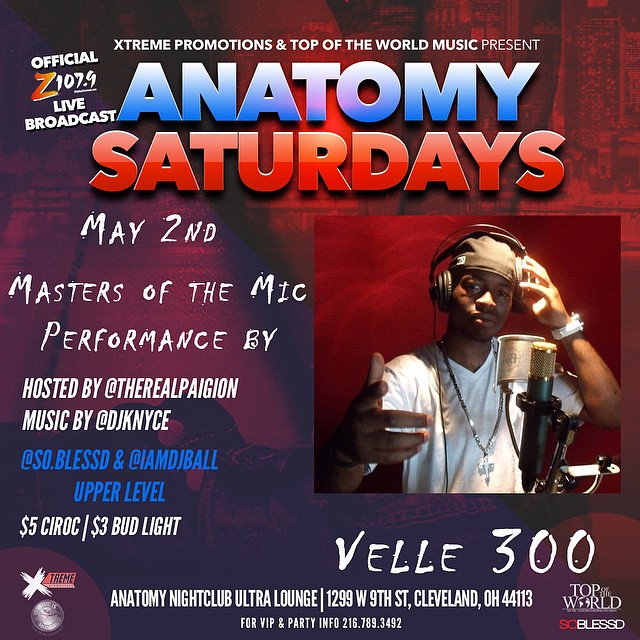The promotional poster for an event titled "Anatomy Saturdays" is vibrant in red, blue, and purple hues. It announces that Extreme Promotions and Top of the World Music are presenting the event, scheduled for May 2nd at Anatomy Nightclub Ultra Lounge, located at 1299 West 9th Street, Cleveland, Ohio, 44113. 

At the top of the poster, blue text reads "Anatomy" with "Saturdays" in red beneath it. There is also a mention of an official Z107.9 live broadcast. The event, "Masters of the Mic," features a performance by Vell 300 and is hosted by @TheRealAbidjan, with music by DJ KNYCE, @SoBlessed, and @IAmDBall. The venue offers $5 Ciroc and $3 Bud Lights. A notable visual element on the right side of the poster is an image of a man in a recording studio, wearing a backward hat, white shirt, chain, and headphones. He is pointing to the camera with one hand while holding his headphones with the other, posing with a neutral expression.

The bottom sections of the poster provide additional details: for VIP and party info, attendees are encouraged to call 216-789-3492. The event seems to be a collaboration involving Extreme Promotions, Top of the World Music, and So Blessed, with Z107.9 hosting a live broadcast.